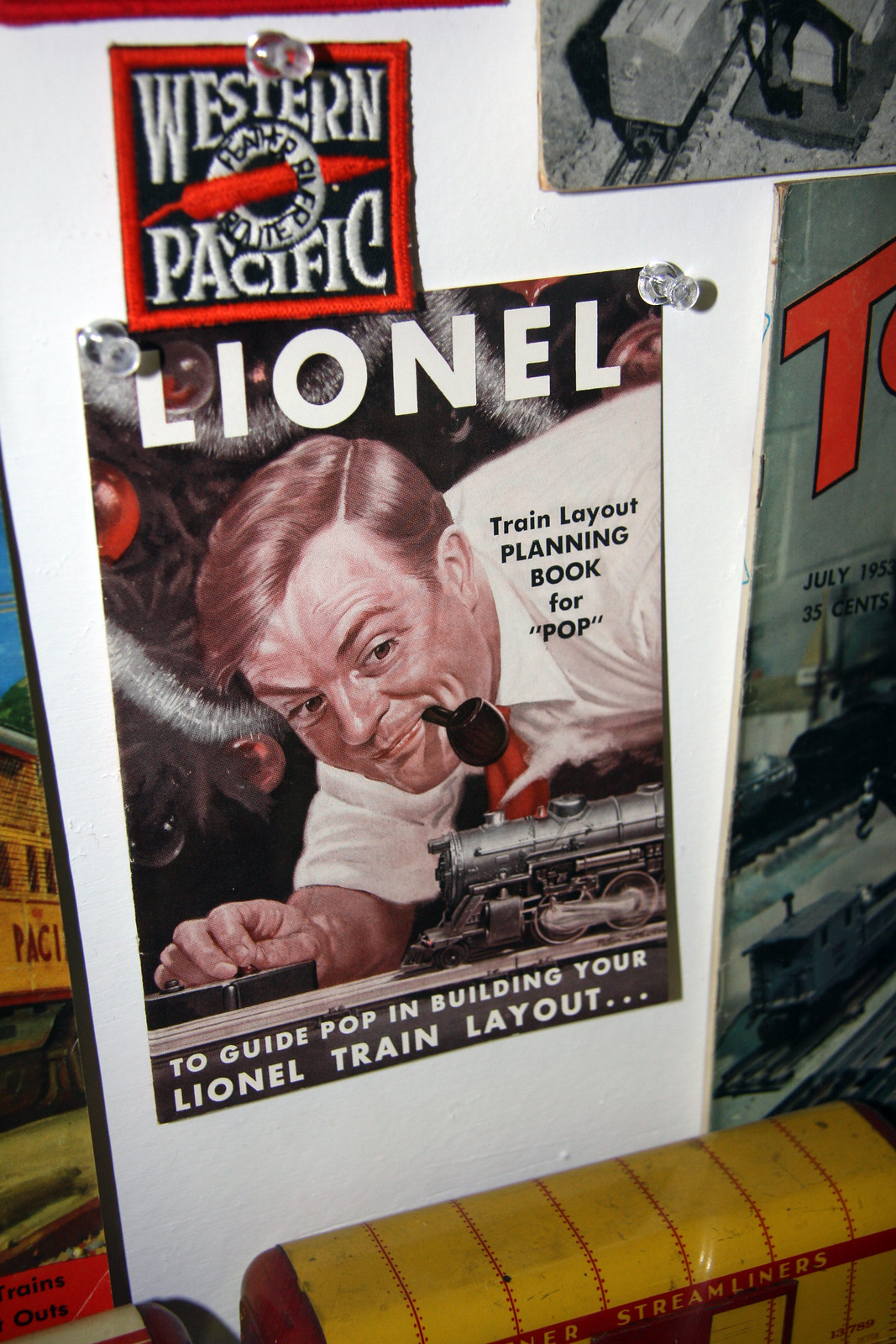The vertically aligned rectangular image features a magazine page pinned to a white surface with clear thumbtacks, likely a whiteboard or wall. The page is primarily an advertisement for Lionel train layouts. At the top of the page, a small square badge with the words "Western Pacific" in white text on a red and black background is visible. Below this badge, two thumbtacks in the upper corners secure the page, which prominently displays the word "Lionel" in large white block letters.

The central illustration on the magazine page shows a cartoon man with short hair, holding a short smoking pipe, leaning down with his arm on the floor. Surrounding the figure is a Christmas tree adorned with red balls and silver tinsel, indicating a festive setting. The text on the page reads: "train layout planning book for pop" and at the bottom, "to guide pop in building your Lionel train layout..." In the lower part of the image, a small section of an old-fashioned steam liner is visible, yellow with red stripes, possibly a toy or train model, against the white surface.